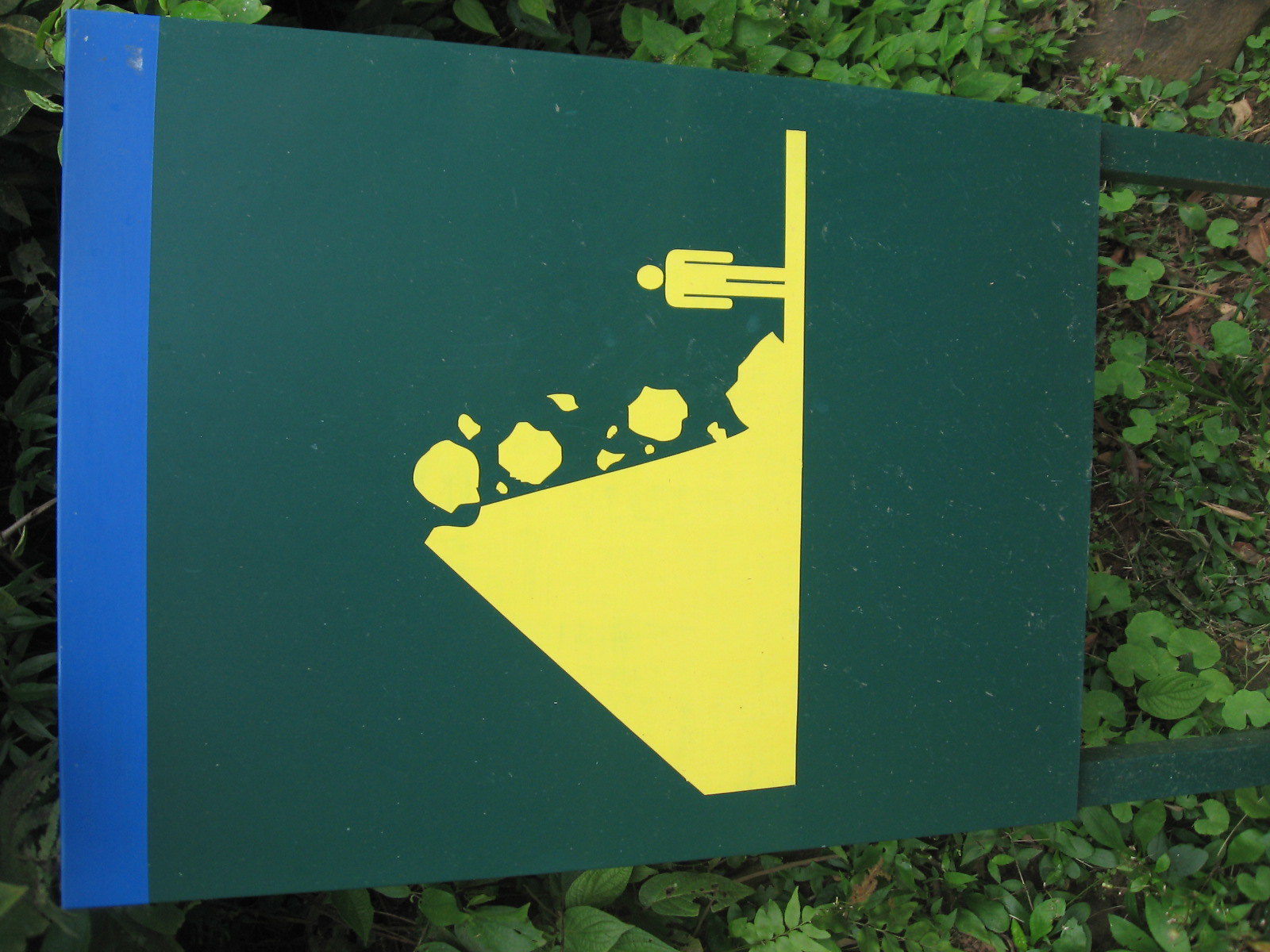In the image, a hunter green wooden sign is depicted immersed in an outdoor scene with dirt and various weeds on the ground. The sign, however, appears rotated, with its base posts, which should be anchored in the earth, positioned to the right. The sign features a vertical rectangular design topped with a strip of medium blue running horizontally along the top 10% of the sign. Dominating the main section is a bright yellow graphic that draws immediate attention. This graphic illustrates a cliff on the left side above a road below, with numerous large boulders or rocks cascading down from the cliff face. At the bottom of the cliff is an iconic silhouette of a person, similar to the figure used on men's restroom signs, standing seemingly unaware of the imminent danger. The purpose of the sign is to warn of falling rocks, emphasizing the potential hazards on the road below.